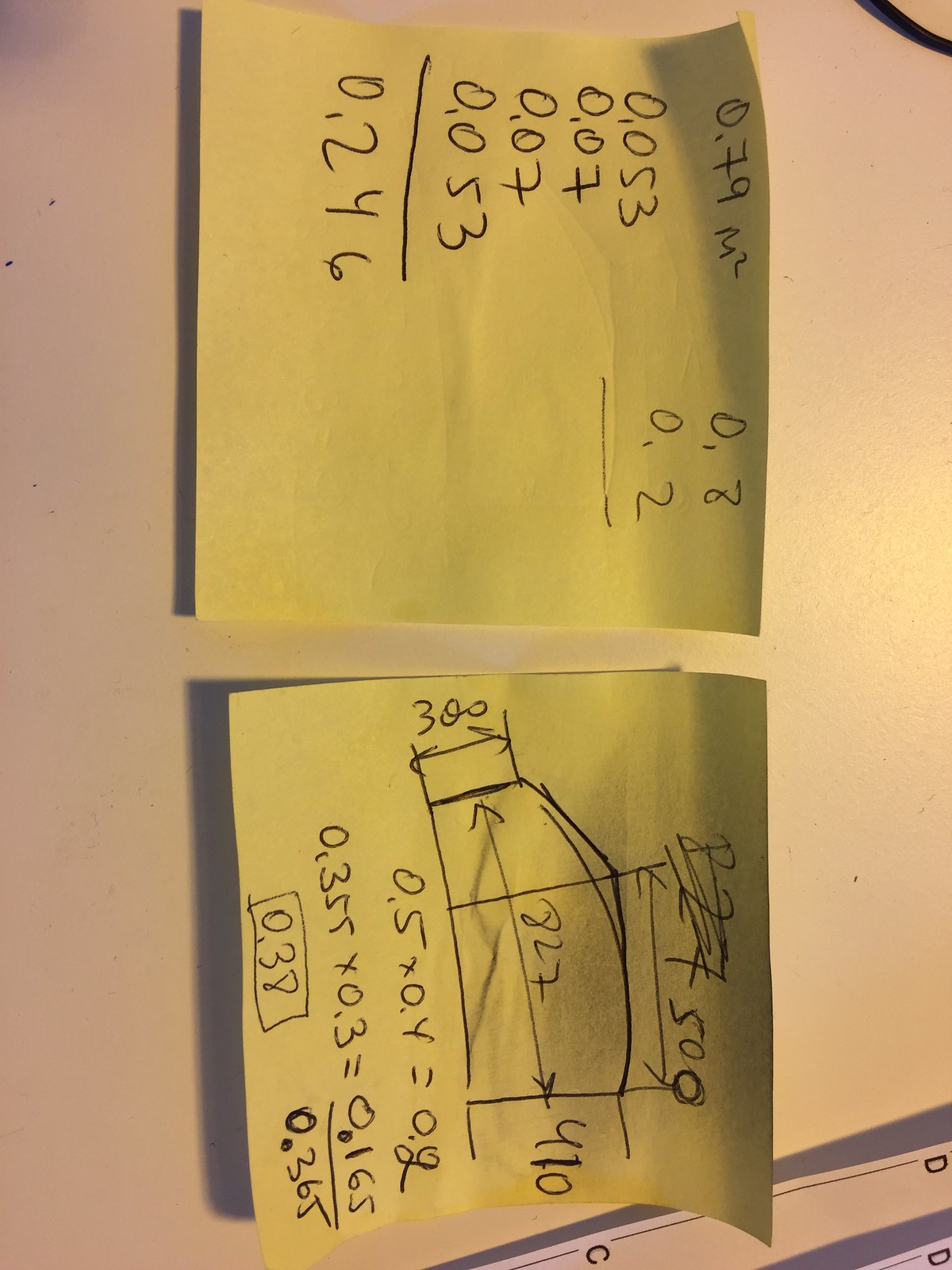This rotated photograph, which is rather dark, features two yellow sticky notes, like those from 3M, that are slightly curled. The first sticky note, positioned towards the top when viewed correctly, contains neatly written numerical values and calculations. It starts with "0.79 M²" on the upper left and continues with "0.8" to its right. Below these figures, it reads "0.053," and off to the right of that, "0.2," both of which are underlined. Additional numbers include "0.07" to the left, repeated beneath, and then "0.053" again, which is outlined. It concludes with "0.246" at the bottom.

The second sticky note, located towards the bottom, appears to have some form of a hand-drawn diagram or sketch with dimensional annotations. The measurements "300," "872," and "410" are inscribed next to corresponding dimensions of the drawing. Below this sketch, there are various numbers and what appear to be equations or additional calculations scribbled in a somewhat chaotic fashion.